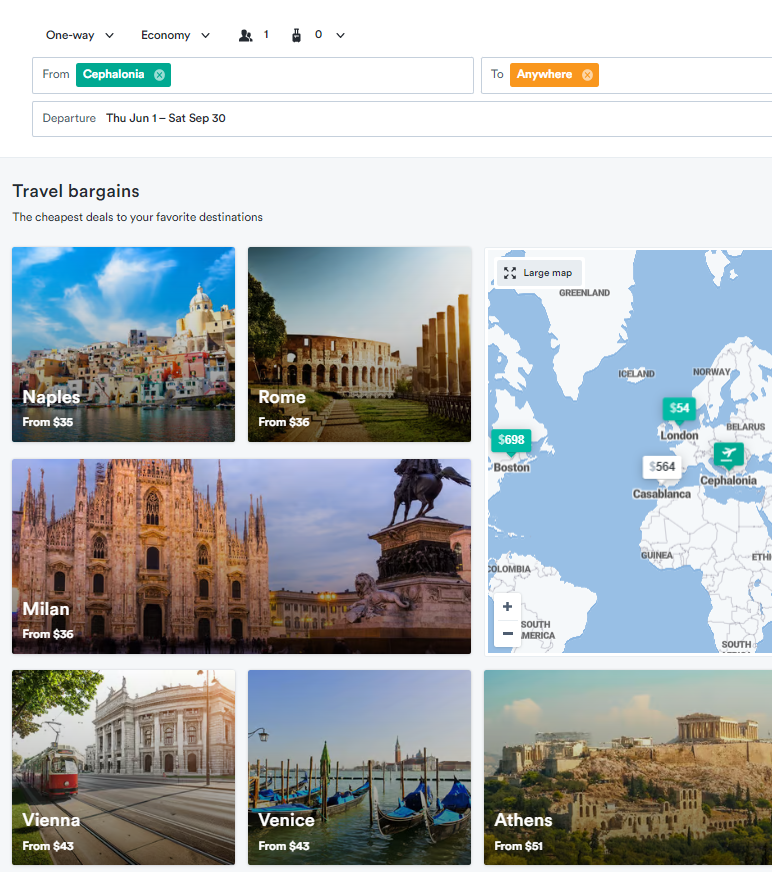A website screenshot showcasing various travel bargains prominently displays attractive deals to popular destinations, with a header stating: "The Cheapest Deals to Your Favorite Destinations." Highlighted offers include:

- Naples from $35
- Rome from $35
- Milan from $36
- Vienna from $43
- Venice from $43
- Athens from $51

A central map visibly includes Greenland, England, and Boston but predominantly features locations near England. The top section of the image includes options for "One Way" or "Economy" travel. Another section indicates offers from Cappellascia between Thursday, June 1st, and Saturday, September 30th.